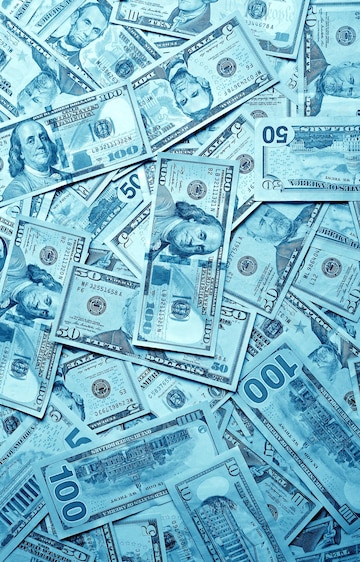This is a detailed color photograph featuring a jumbled assortment of American currency bills ranging from one to one hundred dollars. The bills are lying flat in an overlapping, scattered manner, covering the entire rectangular, vertical image. Among the bills, prominent denominations include one-dollar, five-dollar, ten-dollar, fifty-dollar, and hundred-dollar bills, featuring both newer versions with the distinctive blue security stripe and older ones. The whole image has a bluish tint, making the normally green notes appear blue. The bills are in pristine condition, crisp and unwrinkled, with some facing up and others upside down. The scene is dominated by the higher denominations, especially the hundred-dollar bills, drawing immediate attention. There are no other elements in the image; the focus is solely on the money.